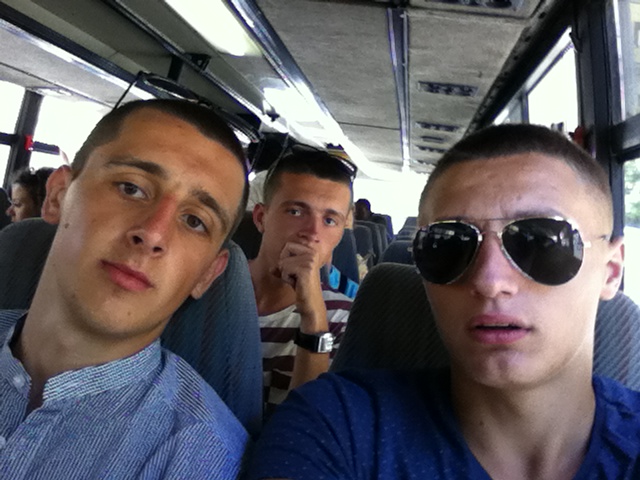This color photograph, taken during the day inside a bus, shows three young men seated in the foreground, all facing the camera. The bus interior features overhead lighting, medium blue seat backs, and windows on both sides. On the right, a man with very short hair is wearing aviator sunglasses and a dark blue t-shirt. To his left is a man with dark hair, clad in a light blue and white striped button-down shirt. Behind these two, between their seats, another man with a short haircut is visible. He is wearing a horizontal black and white striped scoop neck shirt and has a watch on his left wrist, which he is holding up to his face. In the background, the heads of other passengers are partially visible from behind the seats.